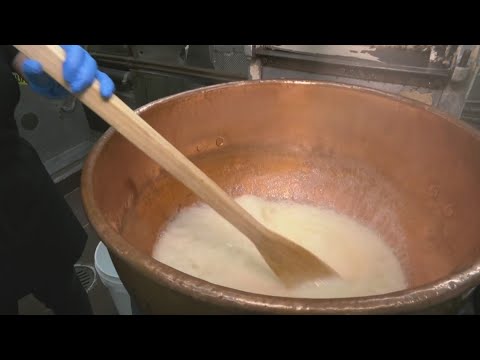The image features a dramatic scene framed by thick black borders at the top and bottom. At the center is a sizable, copper-colored vat, filled to about a third with a frothy, white liquid, potentially a sauce or pudding. The vat is round, extending out of the image boundaries on the right side. A person, predominantly dressed in black, is standing to the left of the vat and stirring the contents with a long wooden spoon, which is approximately two feet in length. The spoon is angled from the upper left to the lower right of the image. Notably, the person has a blue glove on their visible hand that grips the handle of the spoon near the upper left corner of the image. In the background, the setting appears to be an industrial kitchen, with large buckets discernible behind the person. The visual focus and detailed elements collectively create a vivid portrayal of someone engaged in culinary preparation within a professional environment.